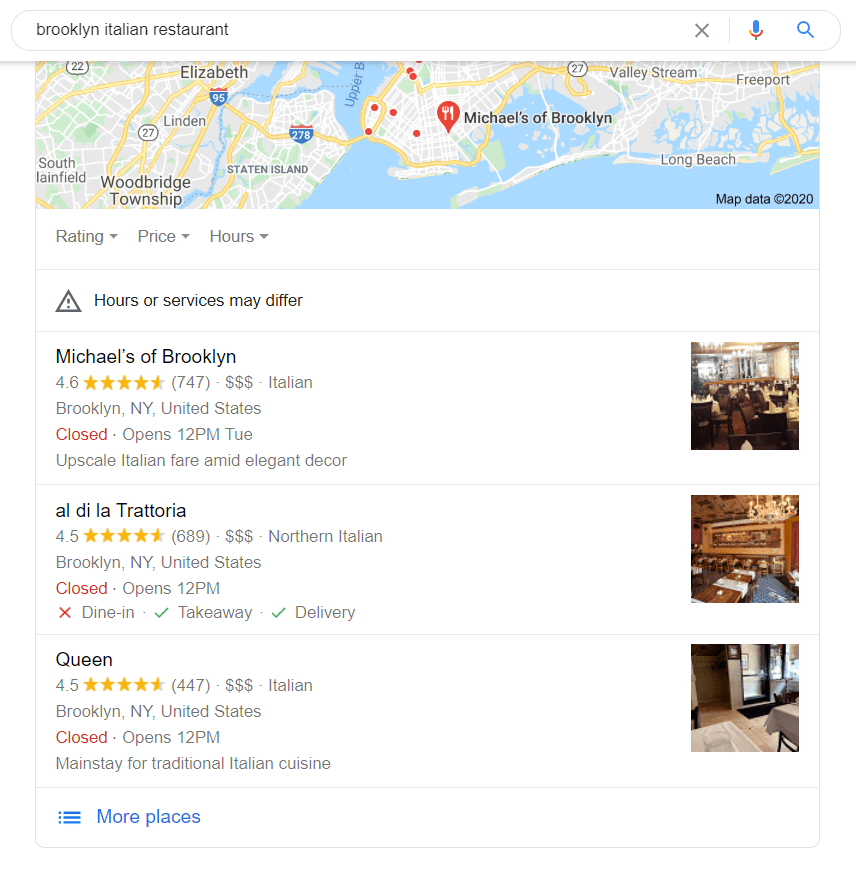The image is a screenshot of a Google search page displaying restaurant details for "Brooklyn Italian restaurant." At the top of the page, there is a large white search bar with a thin gray border. The search query "Brooklyn Italian restaurant" is typed in black, accompanied by a gray "X" on the right side. Adjacent to the search box are a red and blue microphone icon and a blue magnifying glass icon. 

Beneath the search bar, the screen capture shows a Google Maps view indicating the location of a restaurant named "Michael's of Brooklyn." This map features a red location pin, a white fork, and a white knife icon. Scattered red dots also appear on the map. The map includes the surrounding regions, including Staten Island, Woodbridge Township, Valley Stream, Freeport, and Long Beach.

Continuing down the webpage, three sub-menus labeled "Rating," "Price," and "Hours" are visible. Below this, a note states, "Hours or services may differ." The detailed listing for Michael's of Brooklyn displays the following:
- Rating: 4.6 stars based on 747 reviews
- Price: Three dollar signs ($$$)
- Cuisine: Italian
- Location: Brooklyn, New York, United States
- Status: Closed, opens 12 p.m. Tuesday
- Description: Upscale Italian fare amid elegant decor
An accompanying image shows brown chairs and white tables in an elegant dining setting.

Further down, the search results include "Al Di La Trattoria" with:
- Rating: 4.5 stars from 689 reviews
- Price: Three dollar signs ($$$)
- Cuisine: Northern Italian
- Location: Brooklyn, New York, United States
- Status: Closed, opens 12 p.m.
- Dining Options: Dine-in has a red "X," Takeaway and delivery have a green checkmark
An image accompanying this listing shows a wood-paneled dining space.

Lastly, the third listing for "Queen" shows:
- Rating: 4.5 stars based on 447 reviews
- Price: Three dollar signs ($$$)
- Cuisine: Italian
- Location: Brooklyn, New York, United States
- Status: Closed, opens 12 p.m.
- Description: Mainstay for traditional Italian cuisine
The image displayed features tables with simple white tablecloths.

At the bottom, there is a link labeled "More places" in blue with an icon displaying three horizontal lines beside it.